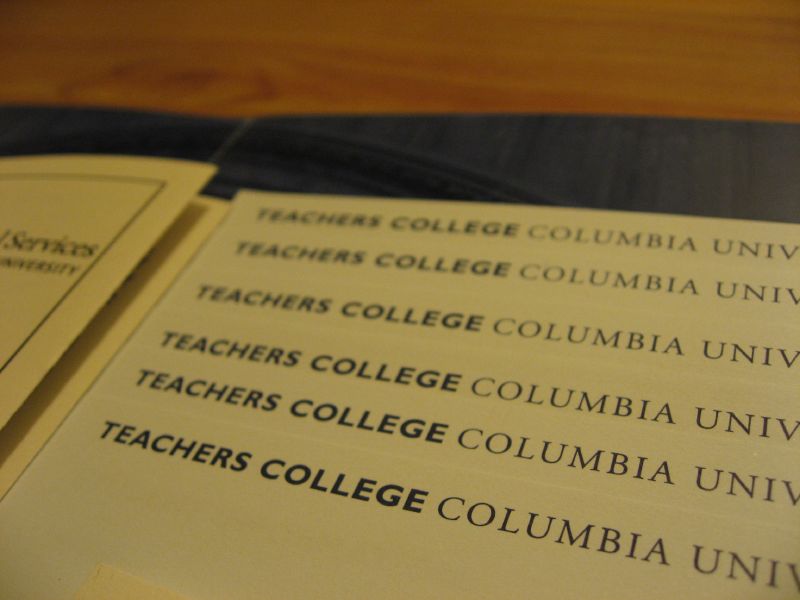This close-up photograph captures a program likely from a college graduation resting on a brown wooden tabletop. At the top of the image, a black or dark blue strip emerges, possibly the spine of a folder or binder holding the program. The program appears slightly disorganized, with multiple pages fanned out and some corners folded down. Centered prominently, the repeated text "Teachers College, Columbia University" is printed in bold blue letters, spanning across possibly six sheets of paper layered atop one another. On the left side of the image, partially visible and slightly blurred, a yellow or tan booklet with the words "Services" and "University" in black text and bordered by a black box line peeks out from the folder. This carefully arranged scene implies a moment of preparation or culmination of academic achievement, distinctly tied to Columbia University’s Teachers College.